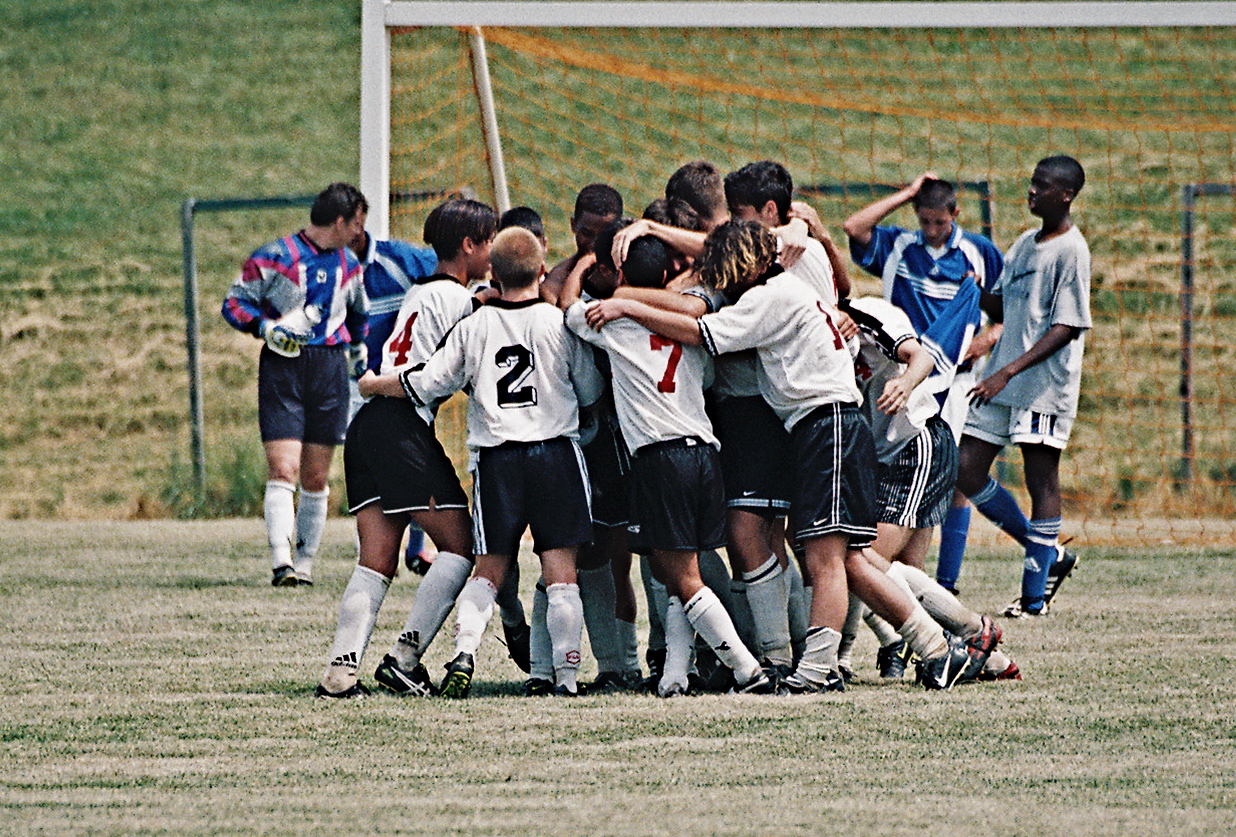The photograph captures a vibrant scene on a lively soccer field featuring a group of young soccer players, likely between the ages of 10 and 12, huddled together in the center of the field. The team, dressed in white jerseys adorned with visible numbers like 2, 7, and 4, paired with black shorts and white socks, appear to be in a moment of either celebration or team strategy. Surrounding the huddle are additional figures—possibly other players, referees, or game officials—some wearing blue tops, one in a gray shirt and shorts with blue socks, who walk near the tall, white goalpost with an orange net. The players' expressions vary, with some smiling, which hints at a celebratory atmosphere, despite the mixed emotions seen on others in the periphery. The field, lush with green grass, is bordered by a grassy hill and three distinctly curved green bars, adding depth and context to this energetic capture of youth sportsmanship.